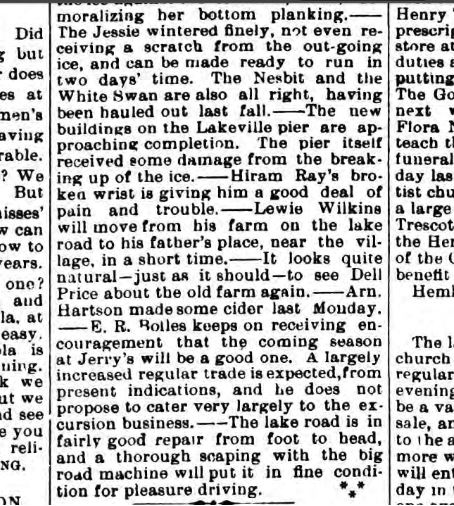The image shows a segment of a newspaper article presented in black text on a white background. The image captures the middle column of the article, with portions of the adjacent columns partially cut off. The text discusses several local updates: it starts mid-sentence stating "moralizing her bottom planking," referring to the vessel Jesse, which wintered without damage from the outgoing ice and will be ready in two days. The article also mentions the boats Nesbitt and White Swan, both of which are also in good condition after being hauled out last fall. New buildings on the Lakeville Pier are nearing completion, although the pier sustained some damage from ice breakup. There's a brief note on Hiram Ray's broken wrist causing him significant pain, and another about Louis Wilkins moving from his farm on the Lake Road to his father's place near the village. Del Price is seen back at his old farm, and Arne Harkson made cider last Monday. There is mention of continued encouragement for the coming season at Jerry's, with an expectation of increased regular trade and minimal focus on excursions. Lastly, it notes that the Lake Road, from its start to end, is in good condition and will be further improved with a thorough road scraping for pleasant driving.